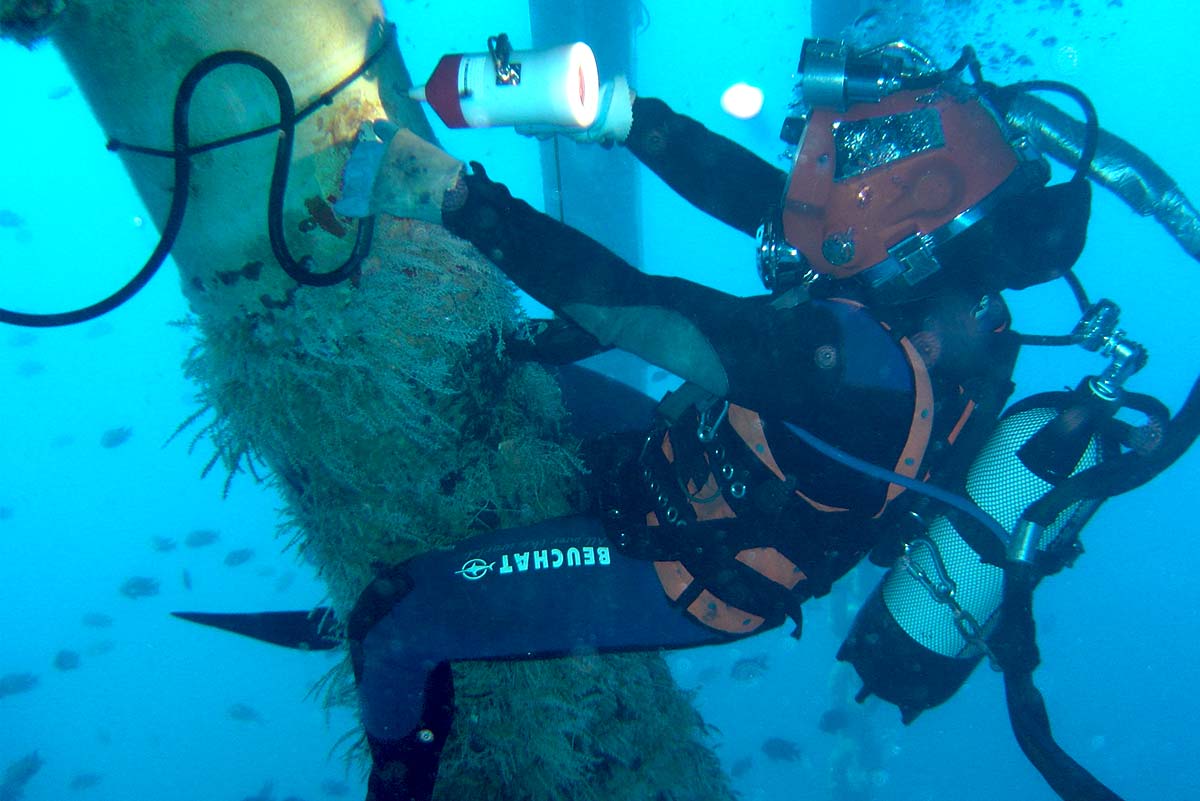In this detailed underwater photograph, set against a striking blue background, a scuba diver is shown actively engaged in an underwater task on a cylindrical, encrusted structure, likely part of a bridge or oil rig support. The diver, clad in a black and orange wetsuit with a distinctive Beauchat logo on his left thigh, is meticulously wrapping a cable around the fibrous growth-covered column. Equipped with protective white gloves, he holds a flashlight in his right hand, illuminating his workspace. The diver has effectively secured himself around the column by locking his knees, ensuring stability in the water. Numerous straps are visible around his chest and abdomen, and a single oxygen tank is mounted on his back, from which extends a substantial hose. Additional gear includes a red helmet and another small hose over his shoulder. Though his face is not visible, the diver's intense focus on the task at hand is apparent. A school of small fish is also present, subtly enhancing the scene's sense of immersion and marine life.